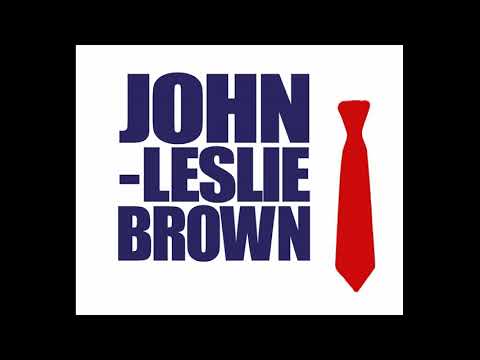The image features a design with a white square background, bordered by a thick black frame approximately an inch wide. At the center of the white background, in large, bold, dark blue capital letters, the name "John-Leslie Brown" is displayed, with each name placed on a separate line. Notably, the word "John" appears thicker and more prominent than "Leslie" and "Brown." Adjacent to the name, on the right side, there is a vibrant red necktie. The high contrast among the colors red, white, blue, and black makes the elements stand out distinctly. The overall setting and style suggest a clean, digital design possibly intended for a political or promotional context.